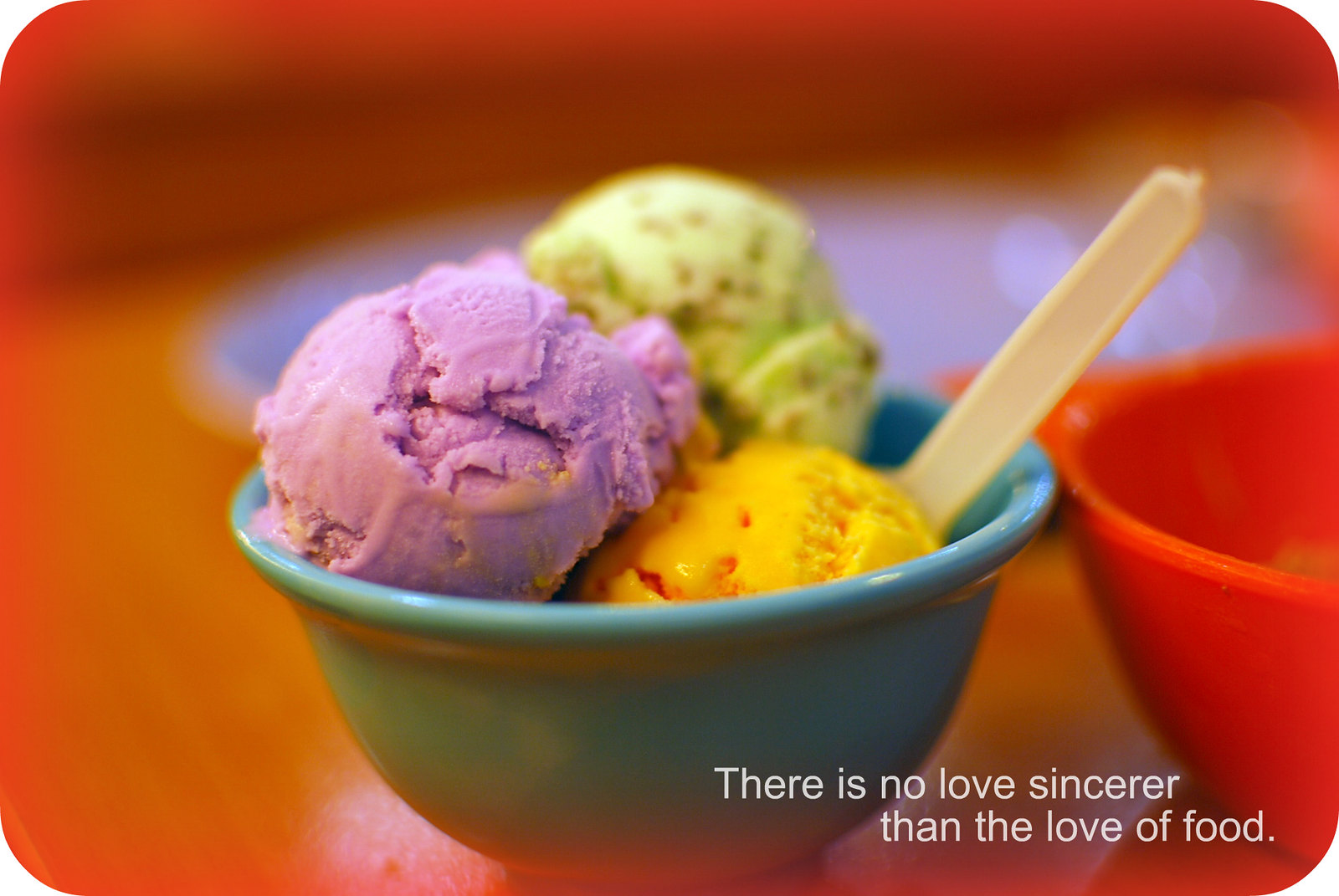The photograph is an extreme close-up shot of a bowl of ice cream featuring three distinct scoops of varying colors and flavors: one purple, one lime green, and one orange. The ice cream is served in a light teal or aqua-colored bowl with a cream-colored plastic spoon sticking out of it. The background of the image is blurry, predominantly featuring mottled swaths of deep red and orange hues, giving it an out-of-focus effect. To the right of the main bowl, a portion of a second orange-red bowl is visible, though its contents are indiscernible. Behind these bowls, partially visible is a purplish plate with a yellow border. At the bottom right-hand corner of the image, white text reads, "There is no love sincerer than the love of food," emphasizing the adoration for culinary delights.